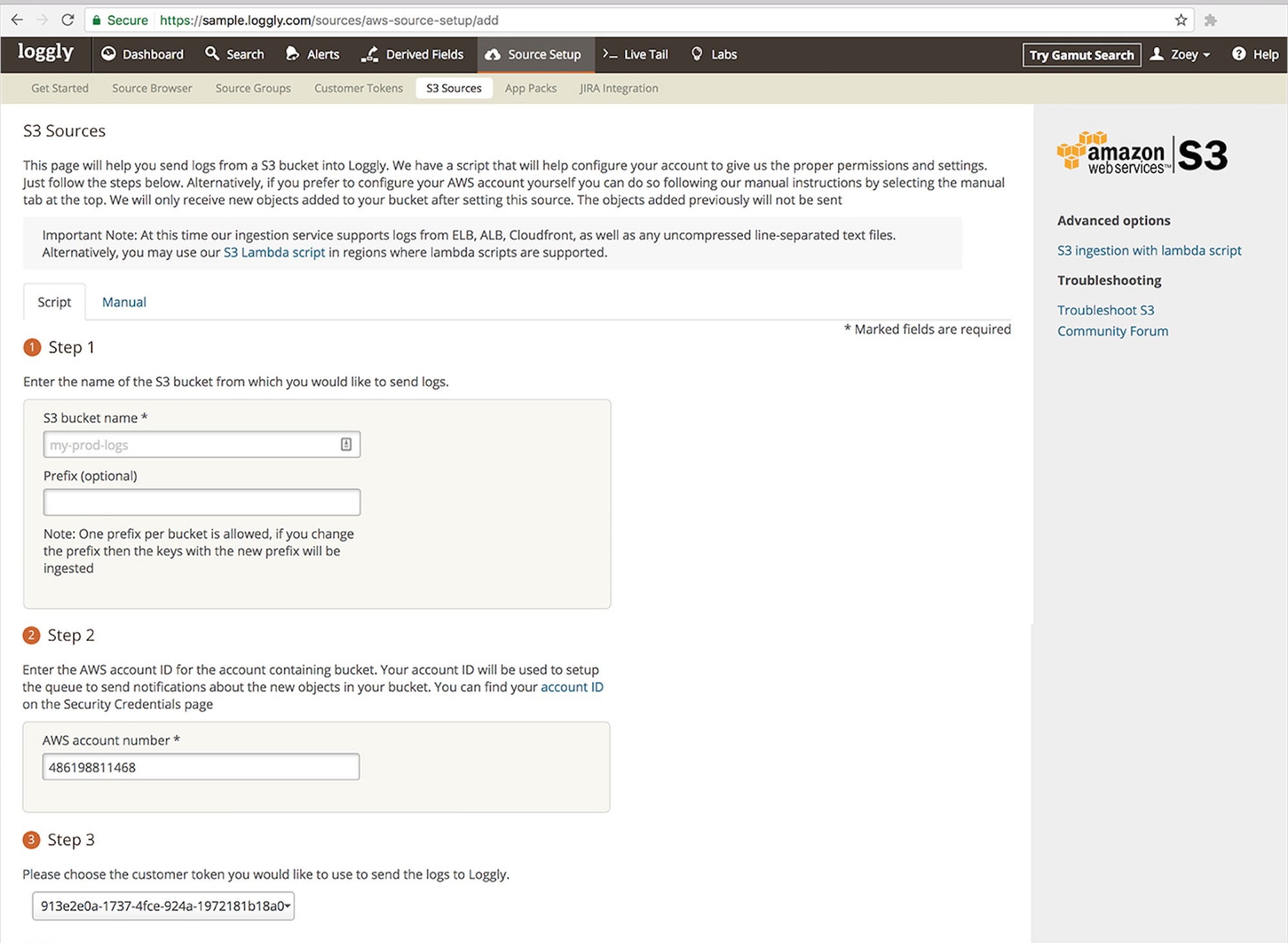The image captures a screenshot of the Loggly website interface. At the top, there is a horizontal brown navigation bar displaying the Loggly logo on the left. Moving to the right, the bar features menu options including Dashboard, Search, Alerts, Derived Fields, Source Setup, Live Tail, and Labs. On the far right, there is an option to 'Try Gamut Search,' followed by a user icon labeled 'Zoe' with a dropdown menu and a Help icon.

Below the navigation bar, the page is organized into various sections. The left column includes options such as Get Started, Source Browser, Source Groups, Customer Tokens, S3 Sources, App Packs, and Jira Integration. Directly beneath the 'S3 Sources' heading is a piece of information with tabs labeled Script and Manual. Additionally, there are three steps sequentially listed as Step 1, Step 2, and Step 3.

On the right side of the image, there is a light gray sidebar titled Amazon Web Services, featuring an S3 icon and the AWS logo.